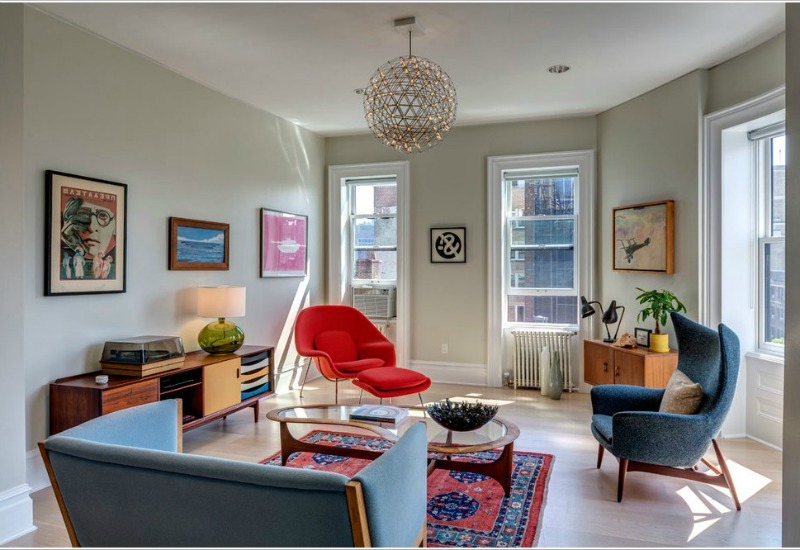The photograph showcases a bright, airy living room characterized by its off-white walls and intricate details in shades of red and blue. The floor appears to be white tile, enhancing the room's vibrancy. Central to the room is a blue sofa paired with a similarly colored, curved-back chair that houses a beige pillow. This seating arrangement is complemented by a glass coffee table resting on an ornate red and blue oriental rug.

On the left wall, an entertainment center made from light wood, reflecting a 1950s design, holds a record player and a lamp with a green glass base. Above this center are three framed artworks: an illustration of a person's face, an ocean scene with clouds in the background, and a third smaller, pink-toned image. Adjacent to this setup is another curved-back red chair paired with a matching red ottoman, positioned strategically between the left wall and a wall that features a window.

The back wall of the room features two large windows with a radiator beneath one and an air conditioning unit beneath the other. Between these windows hangs a fascinating piece of art depicting a round object with a white, squiggly line traversing it. To the right of these windows stands another light wood credenza adorned with a few indoor plants.

On the right side of the room, another blue chair with a beige pillow is placed near a third window, emphasizing the room’s abundance of natural light. In the background, visible through the windows, the presence of other buildings hints at an urban apartment setting.